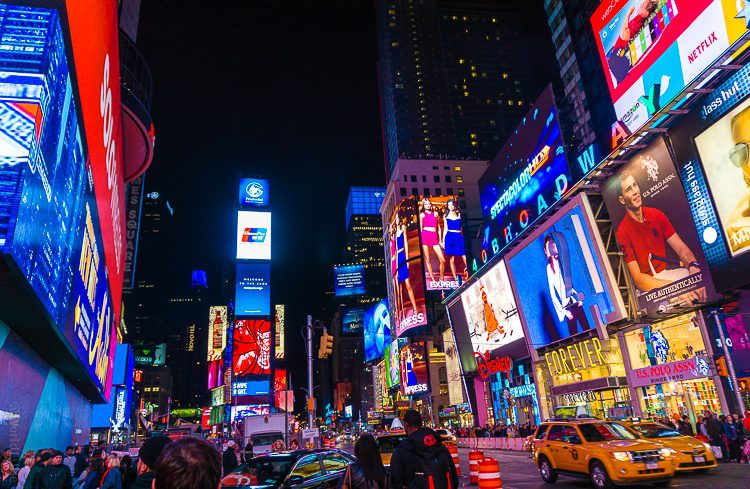The photo captures the vibrant nightlife of Times Square in Manhattan, an iconic urban area known for its dazzling array of advertisements and billboards. Bathed in the vivid blues and reds of illuminated signs, the scene features towering skyscrapers in the background, adding to the night-time splendor. The streets are bustling with a varied crowd, indicative of a weekend evening, yet not overwhelmingly packed. Yellow taxis intermingle with other vehicles, navigating through a somewhat congested area dotted with traffic cones and partially blocked off lanes, suggesting a possible event. Prominent ads from brands like Forever 21, Coca-Cola, and Netflix dominate the scene, alongside promotional materials for Broadway shows. The photograph is taken at an upward angle, accentuating the towering jumbotron screens and making every inch of space appear alive with movement and color.